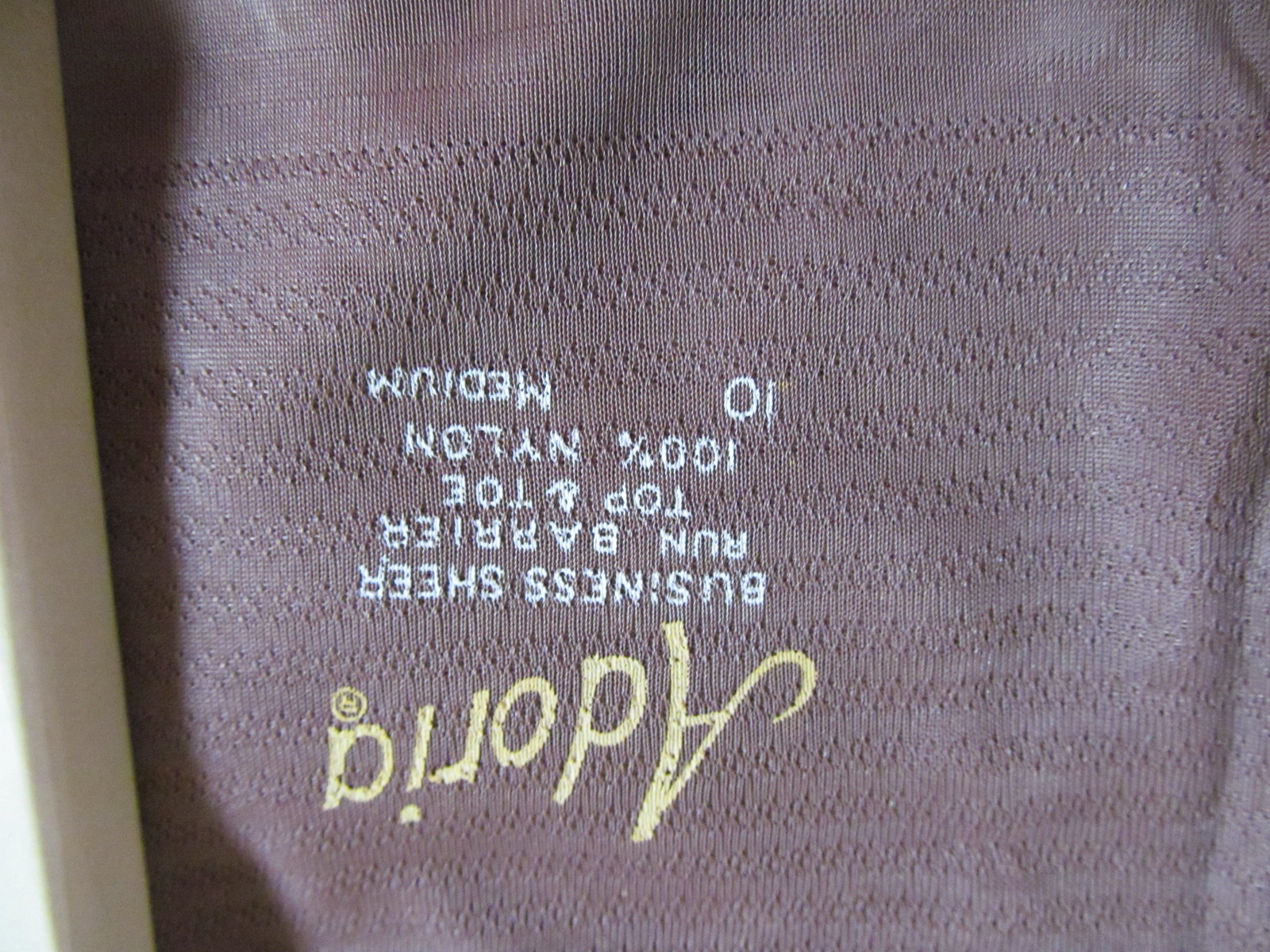The image displays an upside-down label on a garment, which appears to be dark purplish or light brown in color with a textured finish having small lines. The most prominent feature is the brand name "Adoria" stenciled in gold or yellow at the top of the label. Below the brand name, text is stenciled in white, reading "business sheer, run barrier, top and toe, 100% nylon, 10 medium." The garment, potentially either stockings or pantyhose, fills most of the picture. Additionally, a black line runs down one side of the garment, against a background that appears slightly grayish.